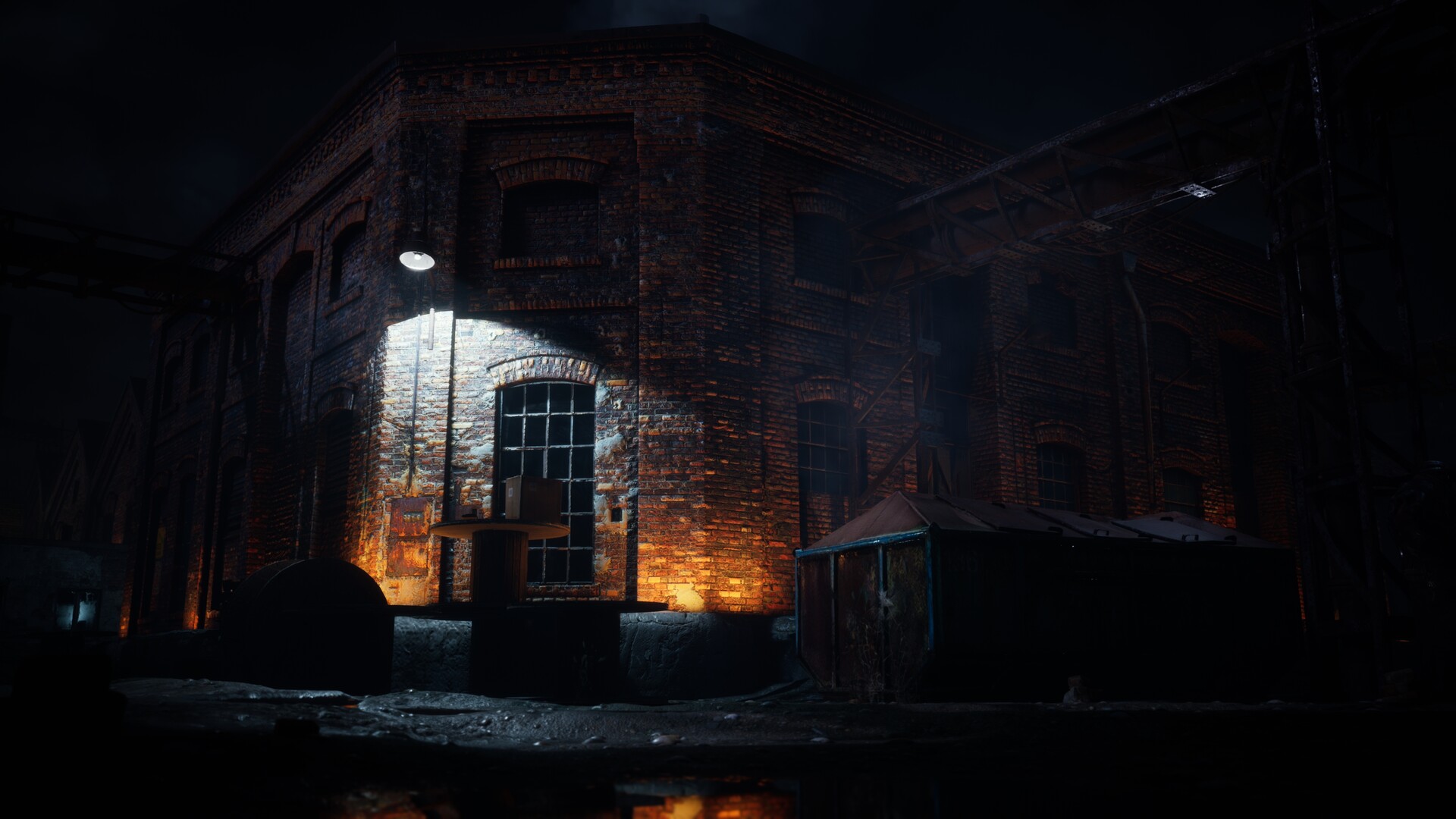The image depicts a nighttime street scene in a city, showcasing an old, seemingly abandoned industrial building made of brick, reminiscent of structures from the Industrial Revolution era. The building, two stories high, stands at the corner of two streets, with a prominent doorway right at the corner that is barred but open to the elements. The scene is dimly lit, primarily by a single overhead light affixed to the building near the door, casting a brownish-reddish hue on the otherwise dark, rundown exterior. Large dark-colored bins, possibly for trash, are visible in front of the building, which appears cluttered and dirty, with some water pooling on the empty street. The ground floor has areas where windows have been filled in with brick, adding to its abandoned appearance. Additionally, a small adjacent tent-like area appears to be closed and unused. A trellis connects this building to another structure just out of the frame, intensifying the industrial yet neglected atmosphere of the scene.